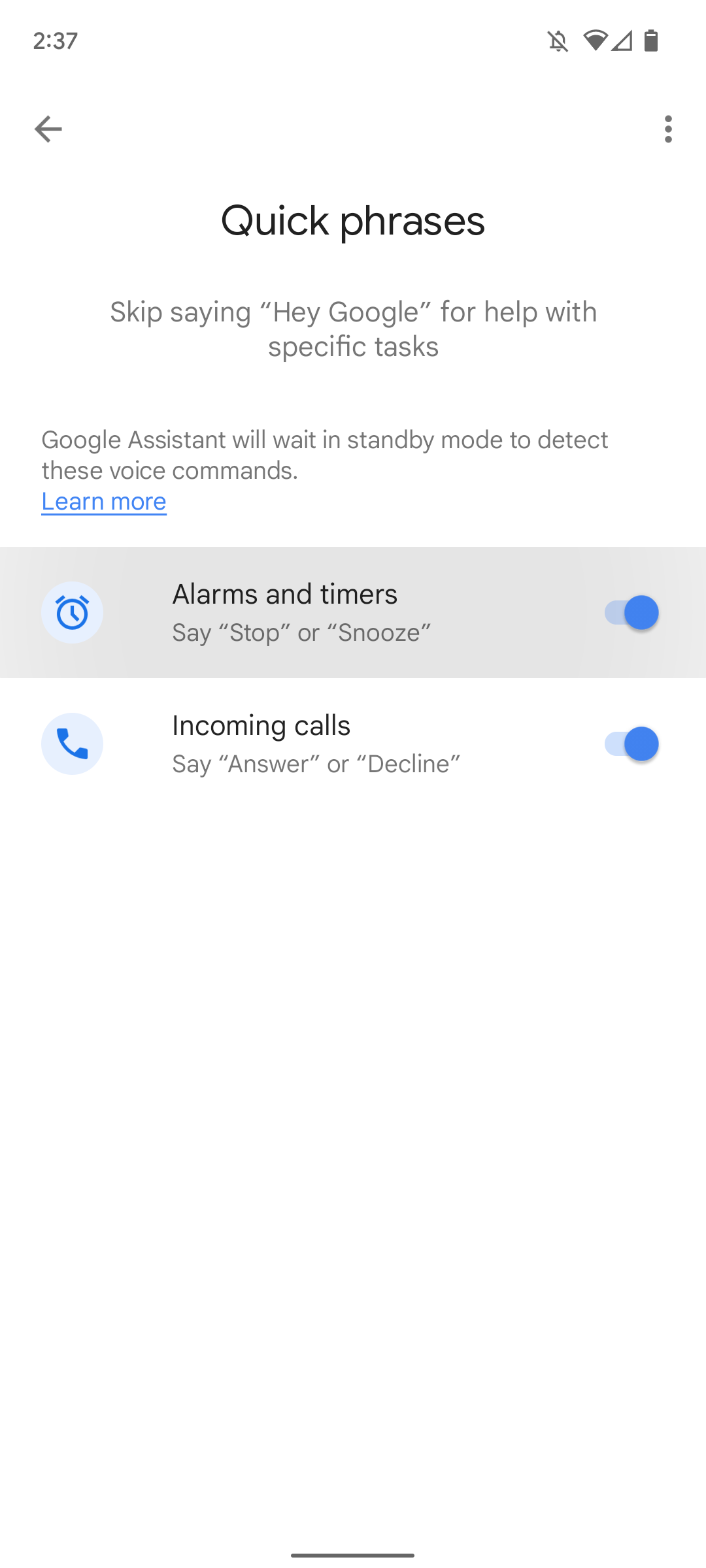This image depicts a screenshot taken on a smartphone, showcasing various Google Assistant settings and functionalities.

At the top of the screen, there is a section dedicated to quick phrases that allow users to bypass saying "Hey Google" for certain tasks. This is highlighted by the text: "Skip saying 'Hey Google' for help with specific tasks."

Just below this phrase, on the left side, there's an informational note stating, "Google Assistant will wait in standby mode to detect these voice commands." Adjacent to this note, there's a blue, underlined "Learn more" link for additional information.

The next section features a gray rectangle containing a clock icon on the left side, illustrating features related to "Alarms and Timers." The instructional text here explains that users can manage these by saying "Stop" or "Snooze."

Further down, another section titled "Incoming Calls" explains that users can answer or decline calls using voice commands like "Answer" or "Decline." This section also includes a phone icon on the left side.

Both the "Alarms and Timers" and "Incoming Calls" features are toggled on, indicated by blue circles situated towards the right of their respective sections. If these features were turned off, the circles would lack color and shift towards the left side.